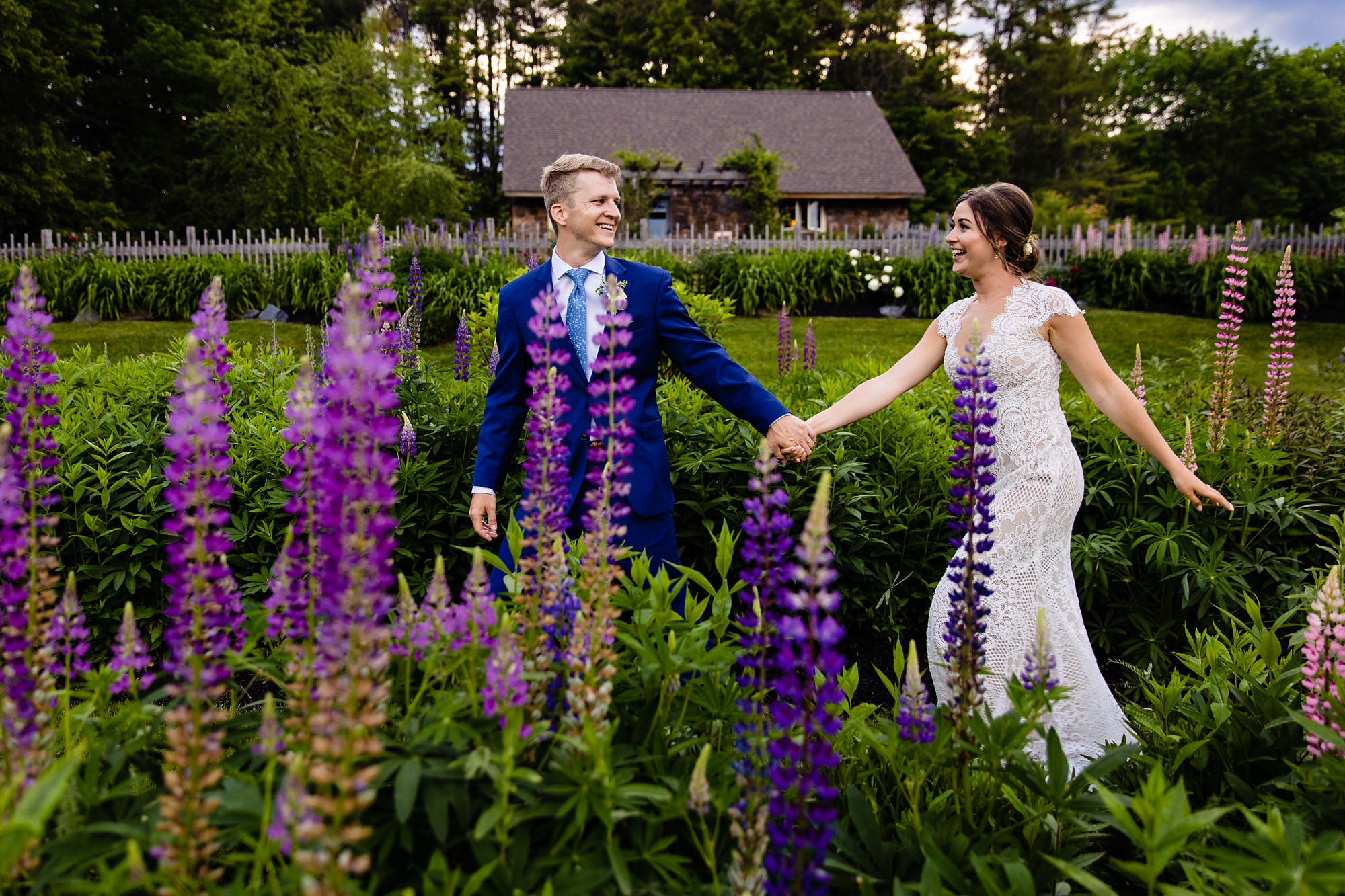In the image, there is a young married couple, likely in their mid-20s, walking hand-in-hand through a lush garden. The woman, who has long brown hair, is dressed in a flowing white wedding gown and is positioned on the right, following the man. The man, who has blonde hair, is on the left and is dressed in a dark blue suit with a light blue tie and a white collared shirt. They are holding hands, with the man looking back at the woman, both smiling warmly at each other.

The garden they are walking through is vibrant and well-kept, with an abundance of lavender plants characterized by their tall, purple flowered stems. Surrounding the walkway are green bushes and patches of grass. In the background, a large house is visible, made of tan, beige, and brown bricks, featuring a dark roof. The house is slightly off-center to the right and is encircled by tall green trees, which frame the scene against a sky of blue and scattered white clouds. A white fence runs across the scene, adding to the charm of the garden setting. The vivid colors of the garden—green bushes, patches of grass, and the purple hues of the flowers—enhance the idyllic moment shared by the couple as they stroll through this picturesque landscape.